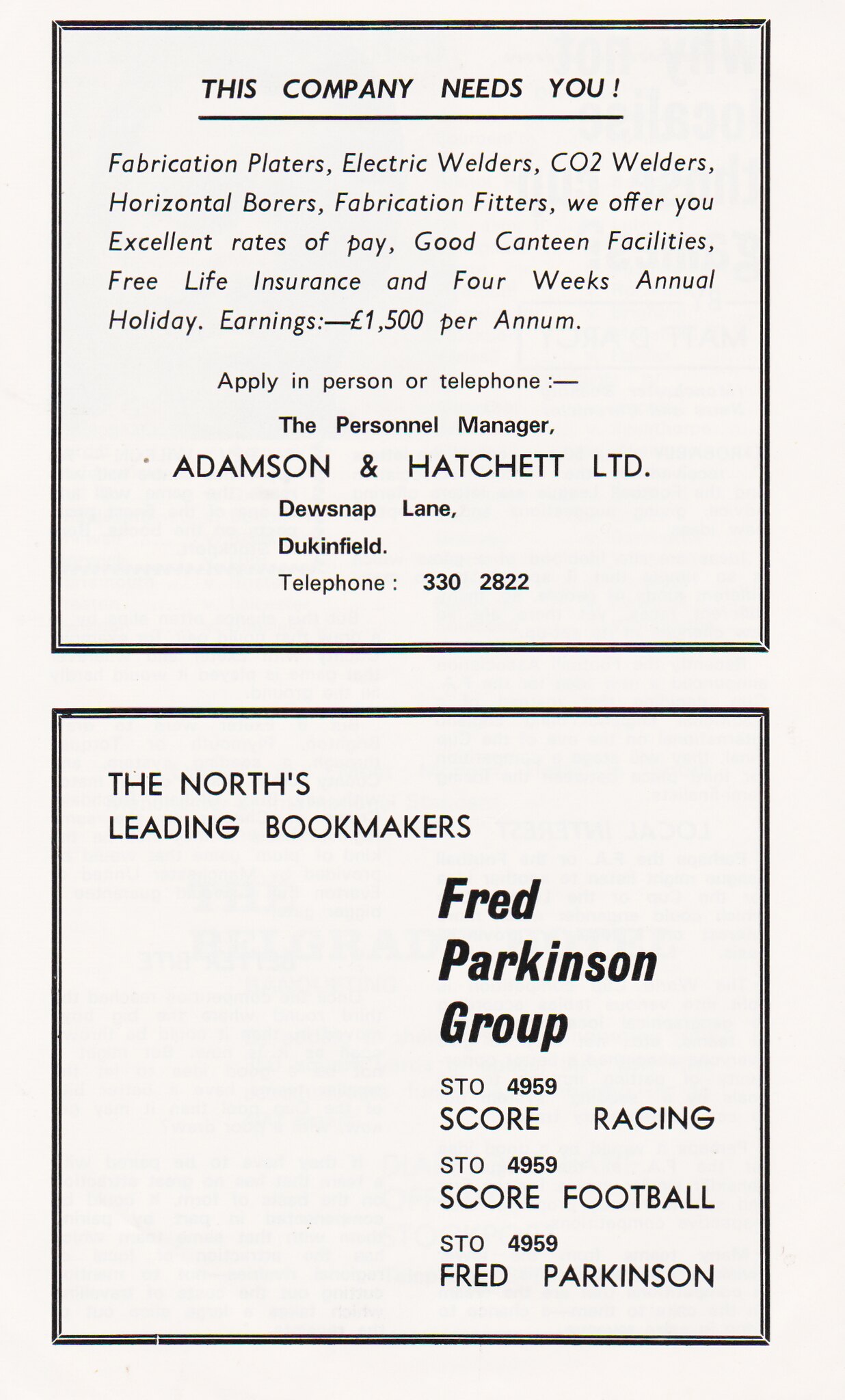The rectangular image, approximately six inches tall and three inches wide with an off-white background, features two equally-sized square boxes arranged vertically, one atop the other. Both boxes are outlined by a thin double-stripped black border and contain black text on a white background.

The top box prominently declares, underlined and centered, "This Company Needs You!" It lists positions available: fabrication platers, electric welders, CO2 welders, horizontal borers, and fabrication fitters. The ad boasts excellent rates of pay, good canteen facilities, free life insurance, and four weeks of annual holiday, with earnings of 1,500 pounds per annum. Applicants are invited to apply in person or by telephone, directed to the Personnel Manager at Adamson and Hatchett Limited, Doosnap Lane, Dukenfield, with the phone number 330-2822.

The bottom box advertises "The North's Leading Bookmakers," the Fred Parkinson Group, listing specific contact numbers: STO 4959 for Score Racing, STO 4959 for Score Football, and STO 4959 for Fred Parkinson. 

Both ads, distinct yet cohesive in design, make for a visually balanced and informative display.